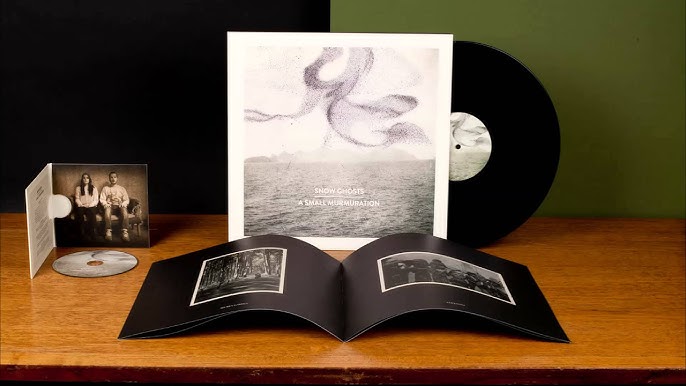A brown wooden table set against a split green and black background holds a collection of band merchandise. An open CD case is positioned on the left side of the table, standing upright with its disc lying next to it. The CD case features an image of two individuals with distinctive long and short hair, both dressed in long sleeves and pants, sitting on a couch. In the center, an open booklet showcases black-and-white photographs framed in white, set against solid black pages. Leaning against the wall is a vinyl LP titled "Snow Ghosts, A Small Murmuration," with its sleeve displaying an artistic design resembling a swirling sky. The greenish olive hue dominates the left half of the backdrop, while the right side remains darker, enhancing the visual contrast in this detailed arrangement of band memorabilia.